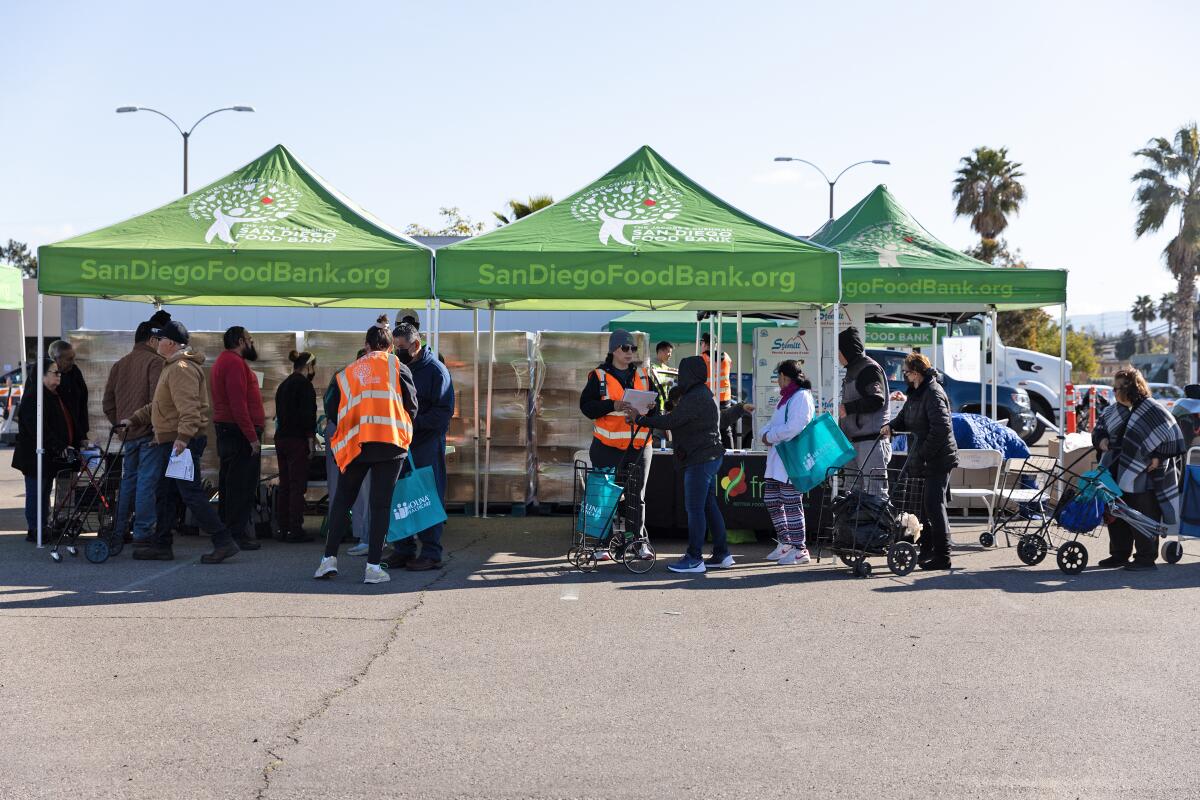This is a detailed photo taken during daylight hours, possibly in a downtown area or large parking lot, where a community event organized by the San Diego Food Bank is taking place. The scene is bustling with activity as people, some with strollers and metal grocery carts, line up to receive assistance. In the background, palm and tropical trees are visible, adding a distinct local feel. The event is set up with three green-roofed tents bearing the sandiegofoodbank.org logo, accompanied by an emblem featuring a figure picking a red apple from a tree.

Underneath these tents, three volunteers donned in bright neon orange safety vests are actively engaged in distributing food and information. They are seen holding green bags and various pieces of paperwork, likely for processing and organizing the event's logistics. Additionally, a stack of boxes can be seen behind the tents, presumably filled with the food items being distributed. This well-organized setup, complete with large lampposts illuminating the area, highlights the collaborative effort to support the community.